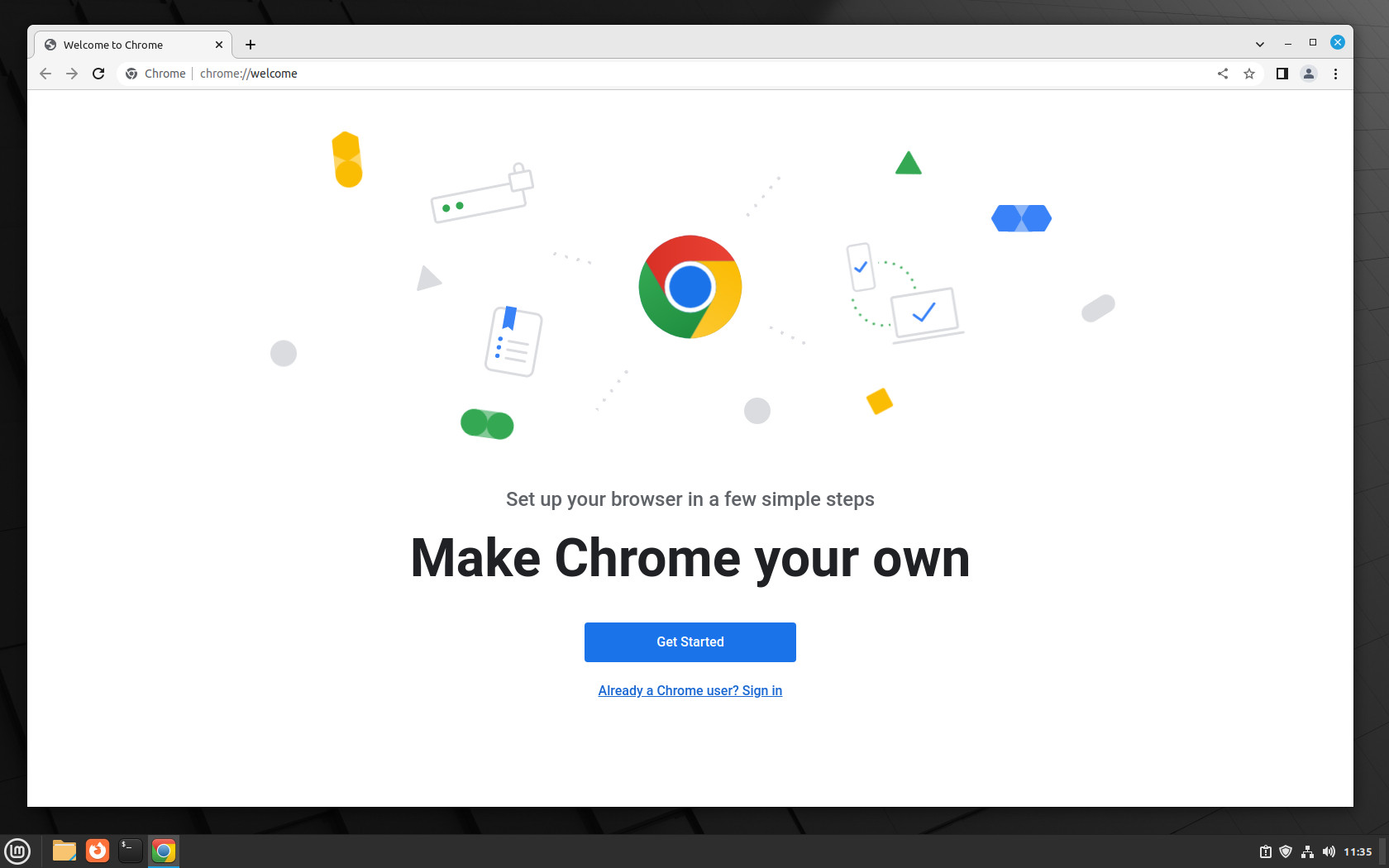This image captures a desktop screenshot displaying an open Google Chrome browser window. At the bottom of the screen, the taskbar is visible, colored in black, with the Chrome icon on the left side indicated as being selected. 

In the active Chrome browser, the user is on the "Welcome to Chrome" page. The page features a clean, white background with the iconic Google logo prominently placed in the center. Surrounding the logo are various playful clipart icons, including representations of a phone, a computer, a bookmark, dots, and triangles, contributing a modern and engaging aesthetic to the page.

Below the Google logo, there is an inviting header that reads, "Set up your browser in a few simple steps," followed by "Make Chrome your own" in a large, bold font, emphasizing personalization. 

Further down, a prominent blue "Get Started" button with white text awaits user interaction, encouraging new users to begin customizing their Chrome experience. Directly beneath this button, a small blue hyperlink text asks, "Already a Chrome user? Sign in," centered to invite returning users to log in.

The browser interface itself appears in a standard gray color, indicating default settings without any personalized wallpaper or themes applied. This minimalistic setup underscores the fresh and uncluttered state of the browser ready for customization.